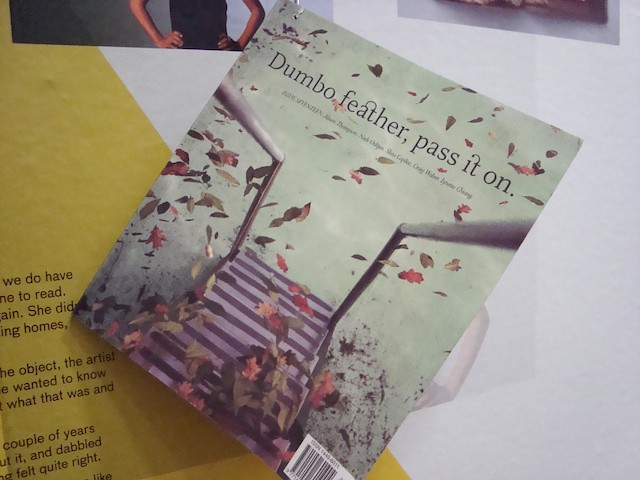The rectangular color photograph depicts the cover of a book or an album titled "Dumbo Feather, Pass It On," displayed against a yellow and white diagonal poster background. The cover itself features an outdoor staircase viewed from above, flanked by two steel handrails. Autumn leaves in shades of green, brown, and orange appear to be floating or scattered across the steps, adding a whimsical touch. Below the main title, faint text possibly listing authors' names is visible, albeit hard to read. A barcode is situated at the bottom right corner of the cover. Above and to the left of the book cover, there are additional images and text partially visible, hinting at a broader collage or display that is not entirely discernible. At the top of the photograph, there appears to be a cut-off image of a woman wearing black with hands on hips. The overall composition suggests a blend of realistic photographic elements and artistic graphic design.